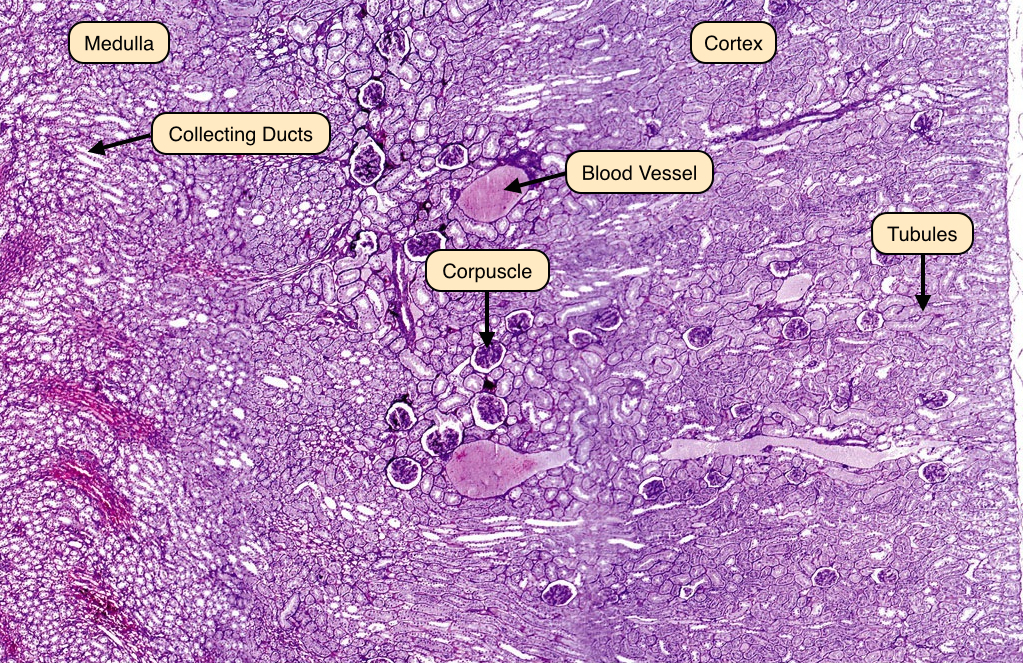The image displays a detailed and colorful microscopic view of blood work, showcasing various anatomical structures dyed in vibrant shades of lavender and purple. The scene, resembling a work of art, features an array of labeled components, each set within beige-colored boxes. Key elements include the medulla labeled in the upper left, with a yellow box and black text indicating "collecting ducts" via an arrow. In the center, a circular structure with a white border is labeled "corpuscle," surrounded by various other cells of differing sizes. On the right side, a purple circle is marked "blood vessel," and additional labels point to "cortex" at the top right and "tubules" with arrows. This intricate arrangement of cells and structures, annotated meticulously, provides a fascinating glimpse into the microscopic world of blood vessels and related components.